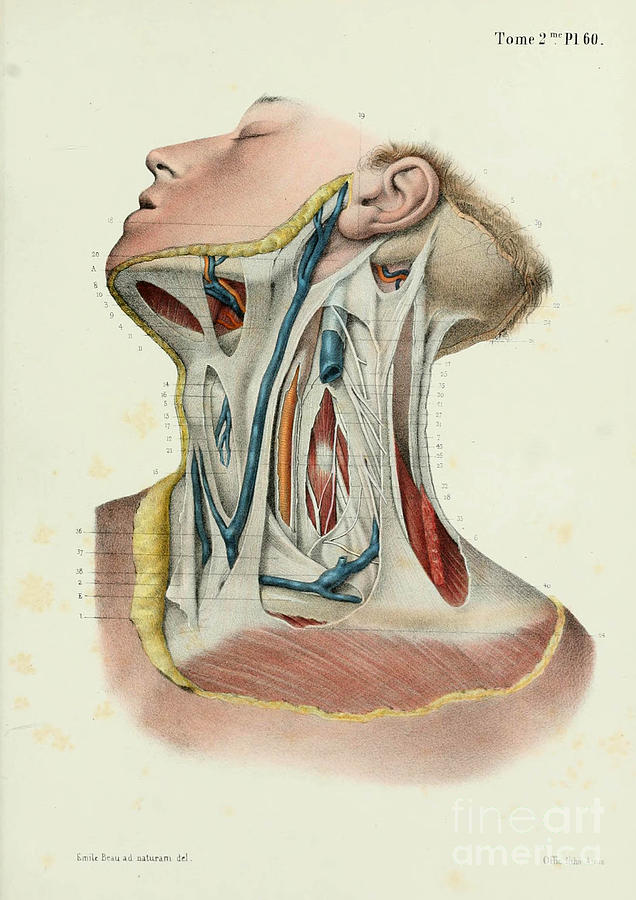This detailed illustration is a cross-section of a human head and neck, presented from a frontal angle. The head is slightly tilted upward, revealing the intricate inner structures from the jaw and chin area down to the chest. The profile displays various anatomical components including muscles, ligaments, tendons, and skin layers, all depicted in vivid colors: black, white, red, orange, and blue. Each part is meticulously labeled with numerous black labels and lines extending outwards, though the text is too small to read clearly. At the top of the image, the text "Tome 2 P 1 6 0" is prominently displayed against a white background, hinting at its inclusion in a detailed volume. In the lower right corner, the image is marked "Fine Art American," indicating its dual purpose as both an artistic and educational piece. The contrasting colors and labeling emphasize the educational value of the illustration, despite some French text and minuscule details that remain illegible.